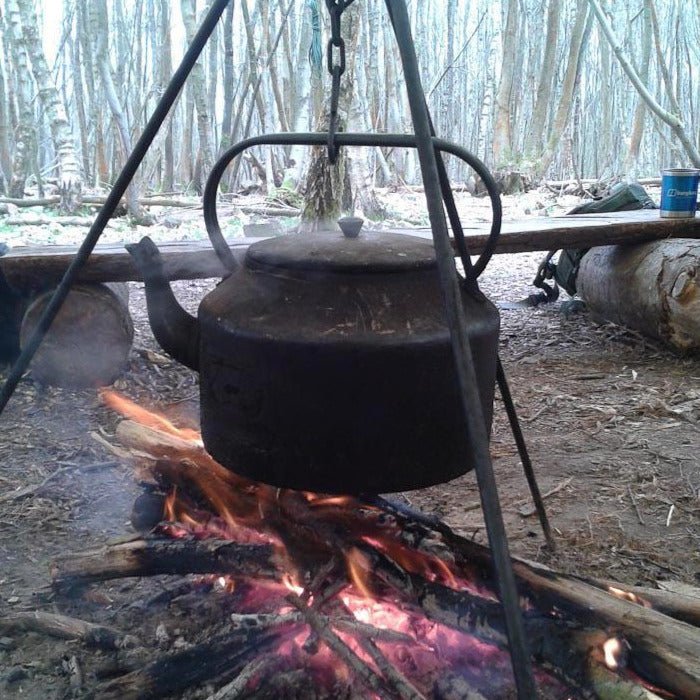The photograph captures a rustic campfire scene set in a forest clearing. At the center of attention is a robust tripod made of steel or metal poles, from which an aged and rusted iron kettle hangs suspended by a chain. The kettle is emitting a steady stream of white smoke or steam, suggesting something is being cooked or boiled inside. Beneath it, the fire burns brightly with vivid red and orange flames, crackling among dark wooden logs arranged to form a stable base. 

In the immediate foreground, two parallel logs serve as makeshift benches, with a wooden plank bridging them; on the right side of this setup, a blue bucket and a green duffel bag rest. The background reveals an expansive forest of tall, slender tree trunks with sparse green foliage, illuminated by bright sunlight that gives the impression of either a snowy ground or a season of bare trees. The overall scene exudes a sense of outdoor adventure and tranquility, emphasizing the rustic and practical elements of campfire cooking amidst nature's serene backdrop.